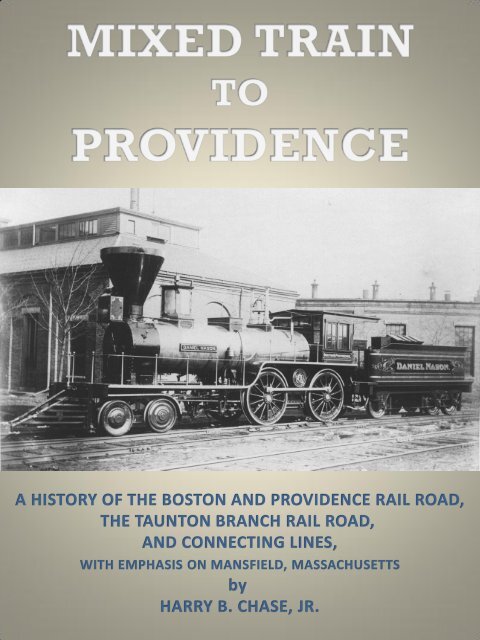The book cover titled "Mixed Train to Providence" features a detailed black and white photograph of an old-fashioned steam engine train positioned in front of a building. The steam train, complete with its characteristic steam stack and visible wheels, has a cart behind it that appears to have the text "Daniel Mason" or something similar inscribed, though the exact name is partially obscured. The primary title, "Mixed Train to Providence," is prominently displayed at the top in white text. Beneath the photograph, the cover reads, "A history of the Boston and Providence Railroad, the Taunton Branch Railroad, and connecting lines, with emphasis on Mansfield, Massachusetts," written by Harry E. Chase, Jr. The smaller text providing additional information is in blue. The overall cover design is colored in shades of gray with some shading to add depth, making both the image and text stand out sharply in contrast.